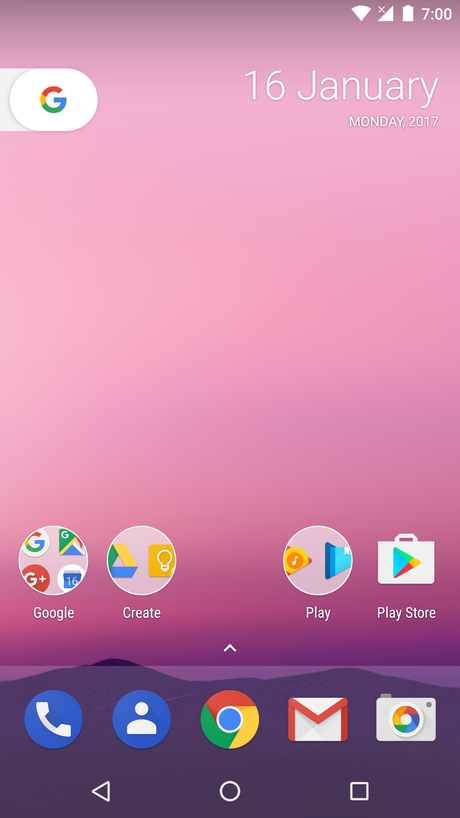This image is a screenshot from a Google phone, taken at 7 p.m. The battery icon at the top right corner shows a full charge. In the top left corner, there's a large "G" icon in Google colors. The background features an ombre gradient transitioning from pink at the top to deep purple at the bottom.

Across the middle of the pink section, four icons are visible. The first icon is labeled "Google," the second "Create," the third "Play," and the fourth icon is a briefcase with a triangle in Google colors, labeled "Play Store." A downward-facing caret indicates additional menu options.

The bottom section of the screen has a purple background with dark shapes resembling mountains. Here, five more icons are displayed from left to right: a phone (likely for calls), a human figure (likely for contacts), the Google "G" logo, an envelope (mail), and a camera icon with the Google colors forming the lens.

Below these icons, there are three navigation buttons: a triangle, a circle, and a square, corresponding to the back, home, and recent apps functions respectively.